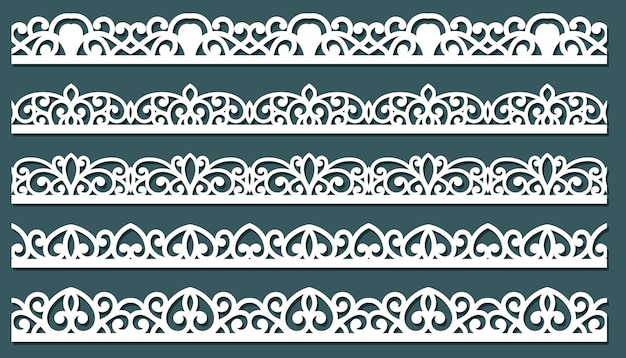This is a computer-generated rectangular image with a sea green background, featuring five distinct rows of intricate white lace or doily-like designs. Each row contains a pattern that repeats itself five times horizontally. 

Starting from the top, the first row showcases a design reminiscent of hearts interwoven with curly cues. The second row features a tighter, more condensed pattern also accentuated with curly cues but less heart-like. The third row, positioned in the middle, resembles a collar adorned with elaborate curly cues. The fourth row suggests botanical elements, possibly leaves and flowers, intertwined with more curly cues. Finally, the bottom row is slightly larger and similar to the fourth, with a design that hints at a fleur-de-lis pattern.

The detailed white patterns contrast sharply with the dark sea green background, making the symmetrical designs stand out vividly.